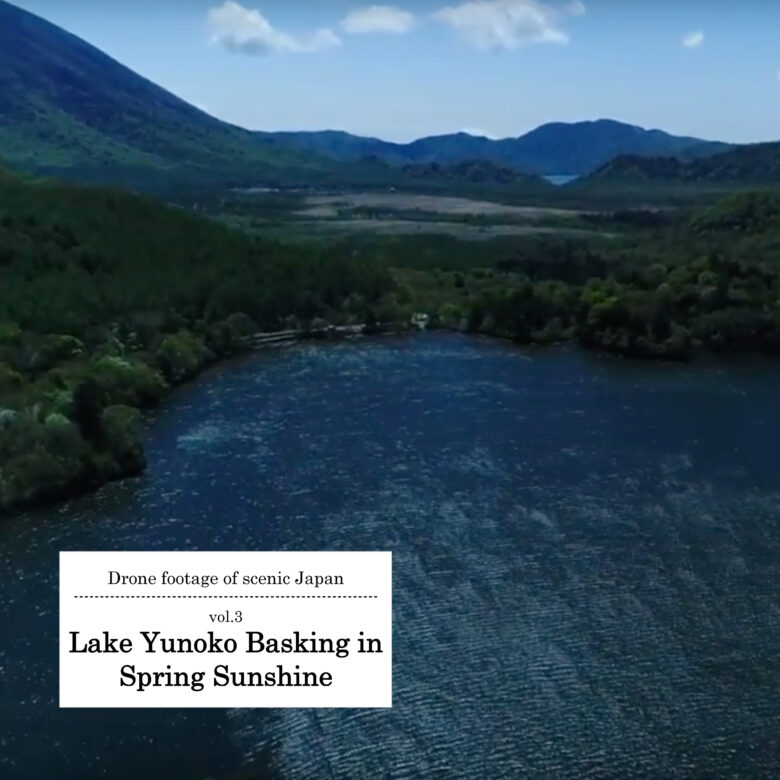This color photograph, captured from a drone, offers a breathtaking aerial view of Lake Yunoko in scenic Japan. The image, part of a series labeled "Volume 3, Lake Yunoko basking in spring sunshine," features a superimposed computerized strip on the bottom left corner that includes this caption in black text against a white background. The foreground reveals the lake's dark blue waters, edged by lush green trees. In the middle distance, more verdant greenery extends, interspersed with patches of brown earth. The upper portion of the photo showcases undulating mountains and hills, with a powder-blue sky dotted with white, fluffy clouds. The entire scene is slightly blurred, lending a serene, dreamlike quality to the snapshot of this spring landscape. Subtle details in the far distance suggest the presence of a building, possibly a caretaker's house, nestled among the greenery.